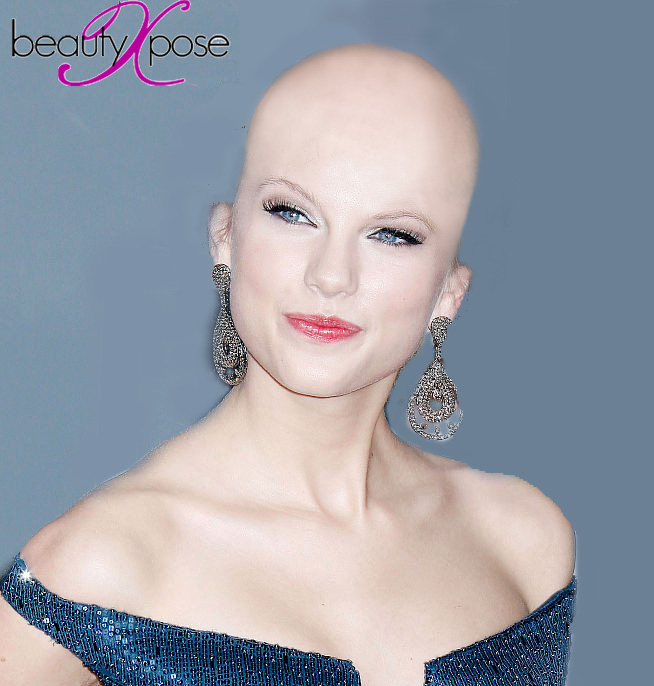The photograph features a confident, bald woman, possibly due to medical treatments like chemotherapy. She has striking light blue eyes and glossy red lips. Her thick eyelashes frame her eyes, enhancing her expressive smile as she gazes in a specific direction. Her bare shoulders highlight a sparkling blue dress adorned with sequins, which glistens against the muted gray backdrop. Dangling from her ears are elaborate, teardrop-shaped earrings encrusted with diamonds. In the top left corner of the image, the phrase "beauty pose" is displayed in a black, lowercase sans-serif font, with a striking magenta "X" separating the words. The combination of her elegant attire and radiant smile suggests she exudes resilience and beauty.